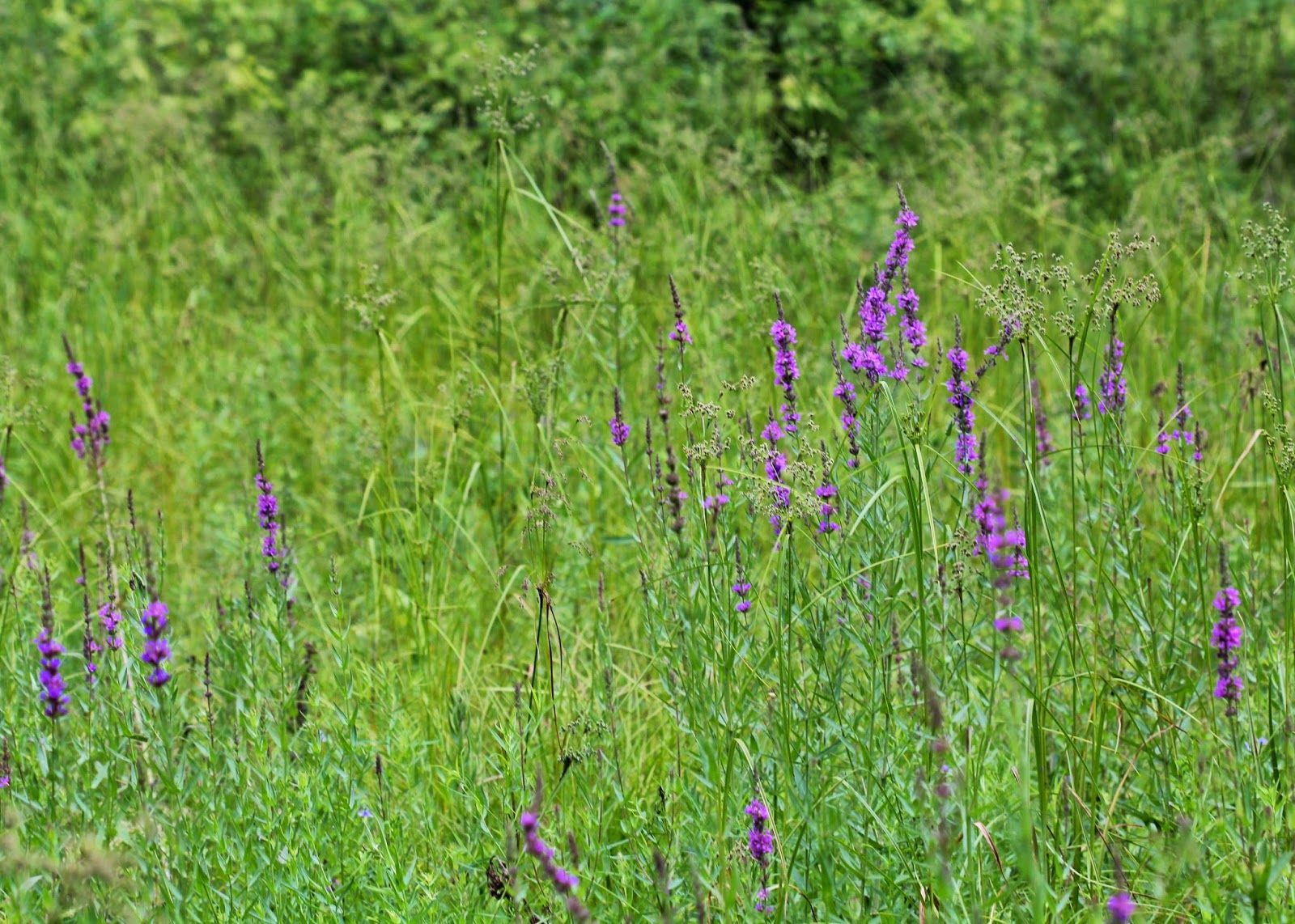The image is a rectangular photograph taken outdoors during the daytime, focusing on a lush, green grassy area. The scene features tall stalks and stems of wild grasses, with clusters of bluish-purple flowers adorning the tops. These flowers have even darker purple centers and a hint of pink, growing in a striking pattern along the stalks. The flowers appear both at the very tips and extending some distance down the sides of the stalks. The greenery occupies most of the image, with a blurred background hinting at green bushes or shrubs. The vivid green wild grasses dominate the foreground, with occasional patches of these distinctive flowers, often resembling fireweed, scattered throughout. The grassy expanse stretches towards the top of the image, with areas of the plants looking ready to come to seed, adding a natural texture to the overall composition. The background bushes provide a dense, leafy border, framing the main subject of the photograph.